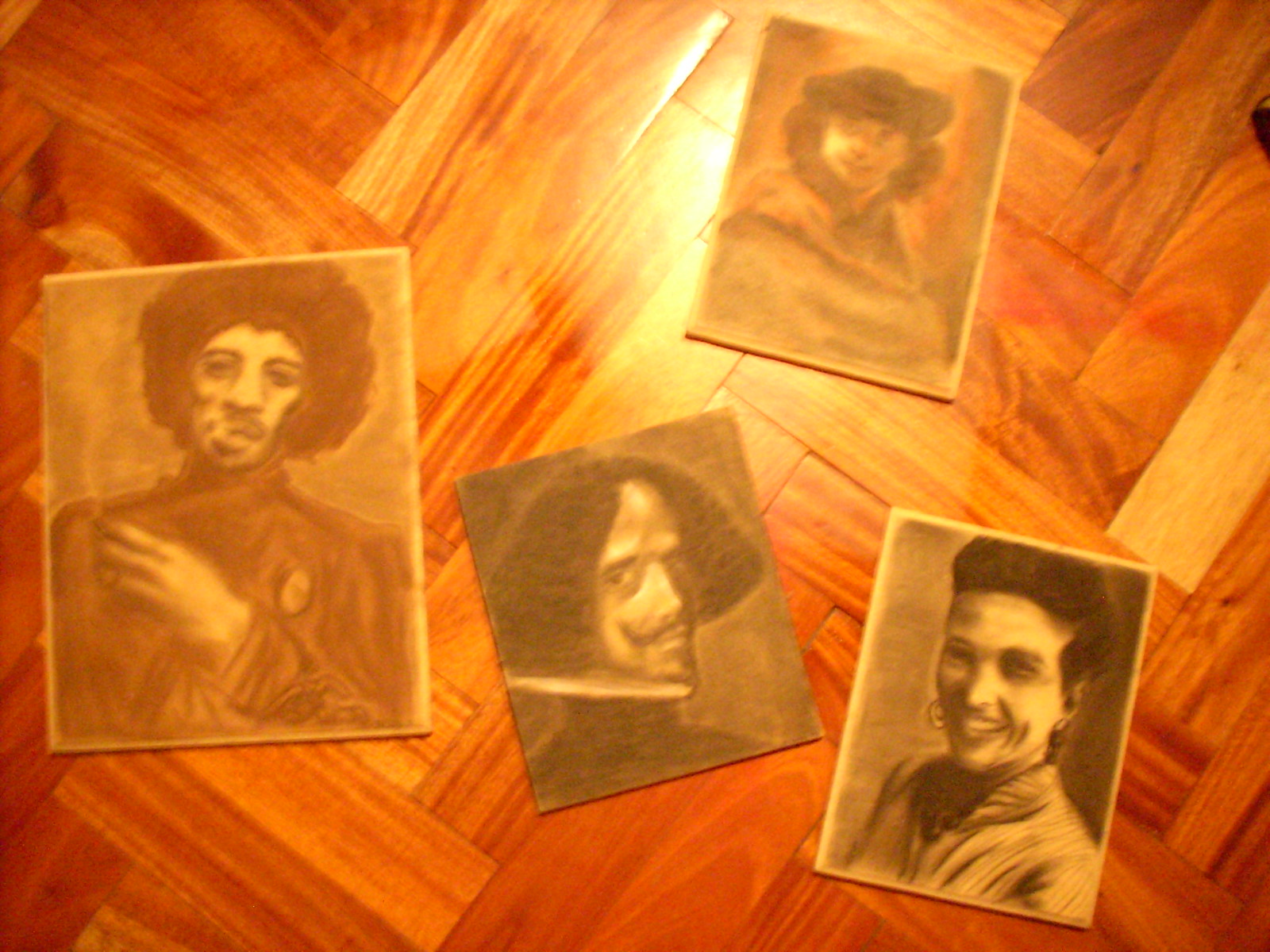The image showcases four monochrome portraits laid out on a medium, reddish-brown, herringbone-pattern wooden floor. Each illustration, approximately postcard-sized except for one slightly larger piece on the far left, features distinct individuals. The first portrait depicts a man with a thick afro hairstyle and a mustache, holding a cigarette and wearing a long-sleeve shirt, his left hand resting on his right shoulder. The second portrays a figure resembling a 17th-century Spanish or French ruler or explorer, with short, thick hair, a mustache that curves upward, and a high white collar—he looks over his right shoulder. The third image features a smiling woman with dark hair pulled back, wearing hoop earrings, a white top, and a beaded necklace. The final portrait is of a woman, possibly from the 1920s, with curly hair peeking out from under a beret and a draped shawl.